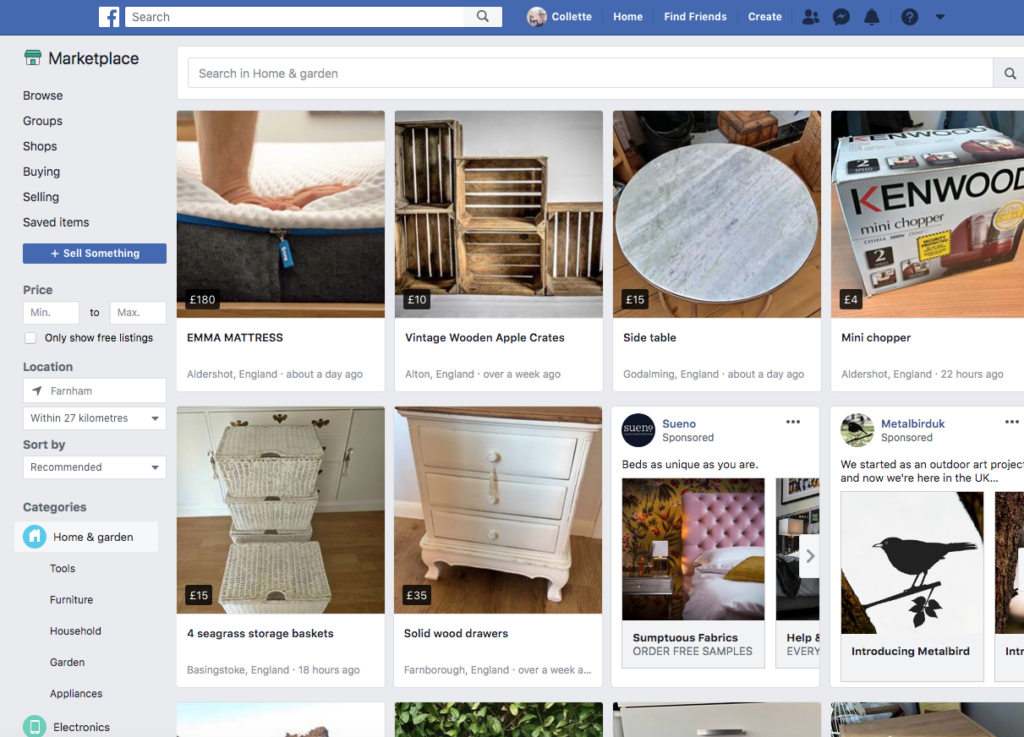The image showcases a screenshot of a Facebook Marketplace page. The top of the page features a royal blue navigation bar that includes the Facebook logo, a search button, and an account icon labeled "Colette." Additional icons present on the bar are "Home," "Find Friends," "Create," and a series of black icons representing two people, Facebook Messenger, a ringing bell for notifications, a question mark for help, and a downward arrow for a dropdown menu.

On the left-hand side, there is a vertical menu beginning with "Marketplace" accompanied by a house icon, followed by options such as "Browse," "Groups," "Shop," "Buying," "Selling," and "Saving" for saved items. Below this menu, there is a prominent blue button with a plus symbol labeled "Sell Something." Further options below, like "Price," include a checkbox for "Only show free listings," and other filters like "Location: Farnham within 27 kilometers" and sorting by "Recommended." Categories listed under it include "Home and Garden," "Tools," "Furniture," "Household," "Garden," "Appliances," and "Electronics."

Centered on the page is a section titled "Search in Home and Garden," featuring a grid of eight images showcasing various items for sale. The first item is a white and gray Emma mattress priced at £180, located in Aldershot, England, and listed about a day ago. Next is a set of vintage wooden apple crates priced at £10, located in Elton, England, and listed over a week ago. A gray side table follows, priced at £15, with its location not specified. After that is a Kenwood mini chopper, in its original packaging, priced at £4. There is also a cluster of seagrass storage baskets and a set of solid wood white drawers priced at £35.

Ending the list, two sponsored ads appear. The first is from Swaino, promoting luxurious beds with the tagline "Beds as unique as you are," featuring sumptuous fabrics and offering free sample orders. The second ad is from Metal Bird UK, which started as an outdoor art project and showcases a black silhouette of a bird on a branch.